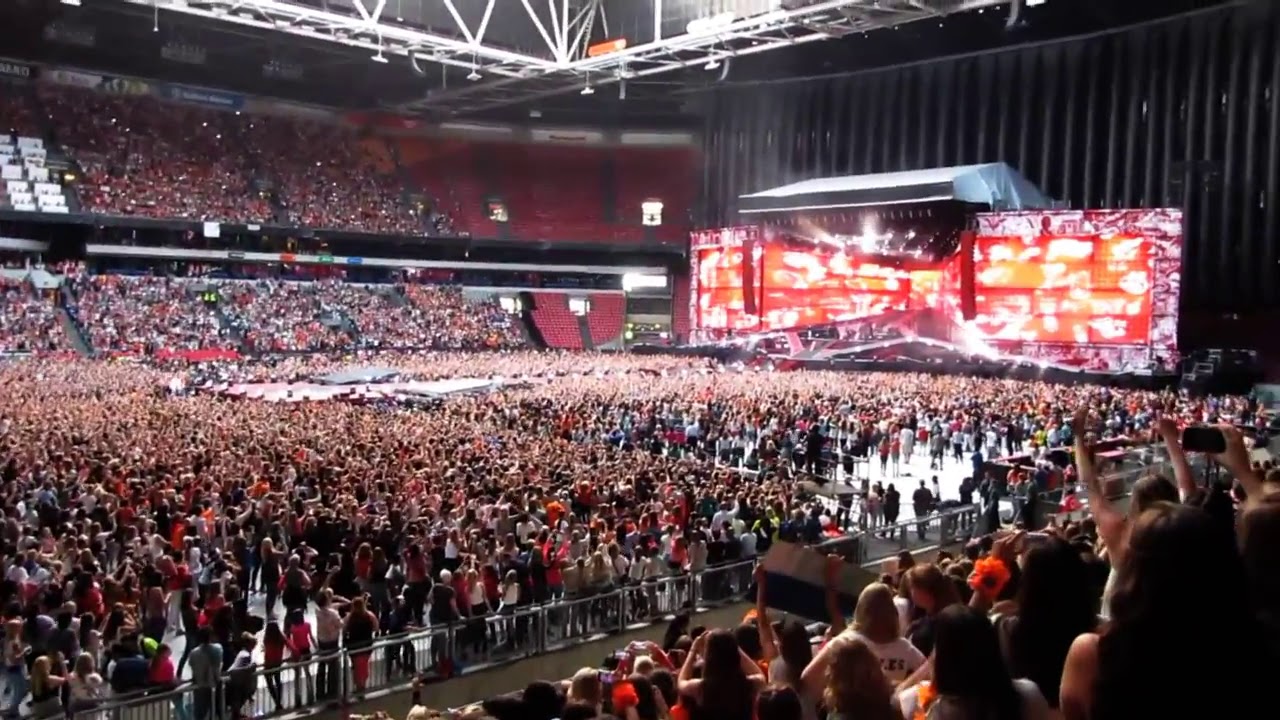The image captures a massive rock or pop concert inside a stadium, which could be a baseball or football arena. The entire stadium is packed with tens of thousands of cheering fans. The pit area in front of the stage is densely filled with people standing, while the bleachers are also crowded with spectators.

The stage stands in the center and features an array of lights and massive screens. One prominent screen toward the back displays vibrant, dynamic orangey-red designs that appear three-dimensional. Above this screen is a large vent. The stage itself is set against a backdrop of black curtains. Numerous colored lights (orange, yellow, purple, blue, and green) illuminate the venue, with some of these lights directed toward the screen.

Suspended from the stadium’s closed ceiling are metal bars likely used for camera equipment and other technical setups. There is a small circular gap to the bottom right of the center of the view, the only section not densely packed with people. Although no performers are visible, the flashing lights suggest the concert is either about to start or is already underway.